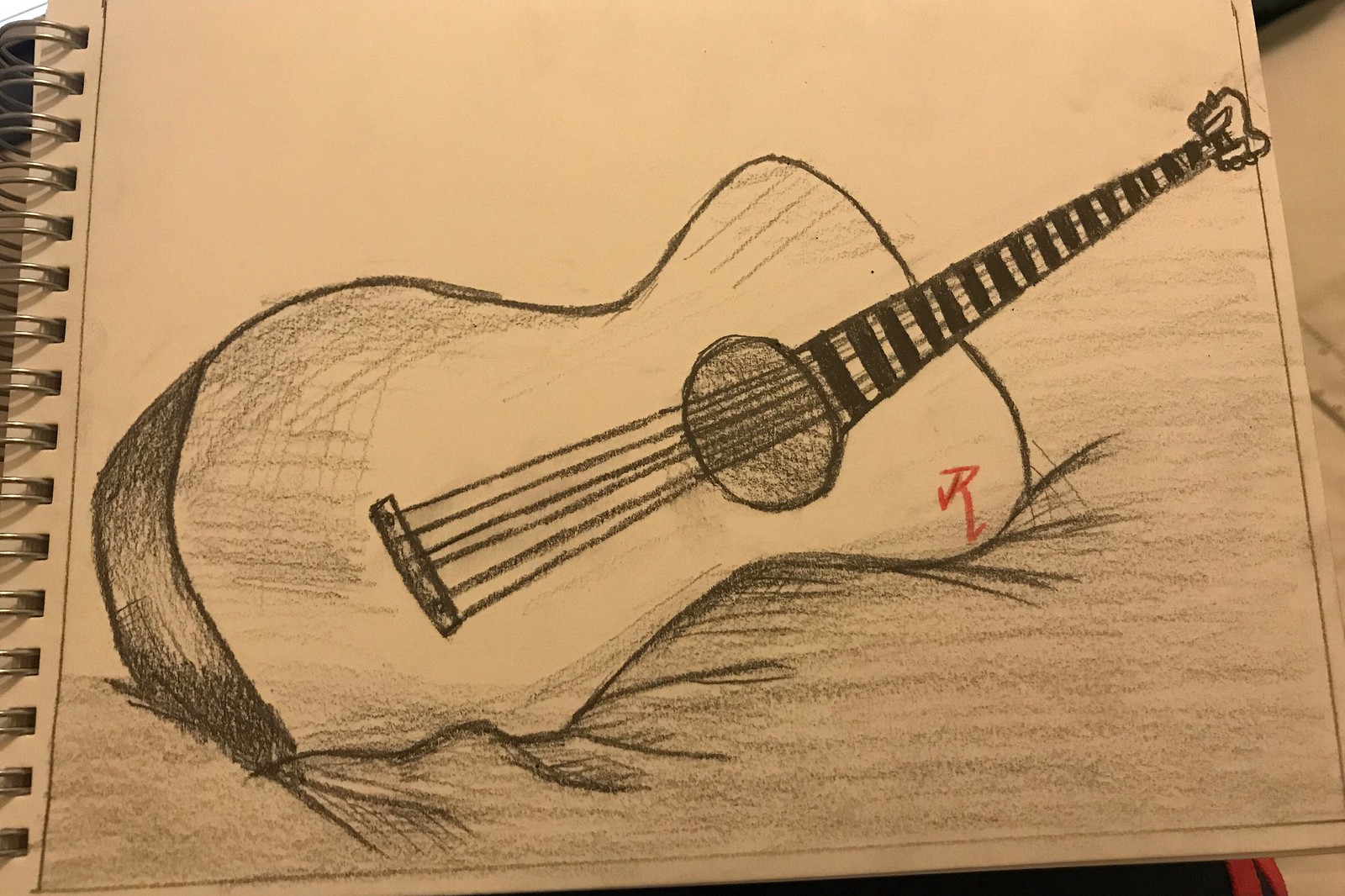The image captures a detailed pencil drawing on a spiral-bound notebook, where the spirals are clearly visible on the left side. The primary subject of the drawing is an acoustic guitar, depicted as partially emerging from a mound of dirt or soft material, with the body of the guitar embedded into the ground and the neck extending towards the top right corner of the page in a diagonal orientation. The guitar handle features black stripes running vertically along its length. Notable shading is applied to the bottom end of the guitar and the surrounding mound, giving the drawing depth. A distinctive red letter 'R' is marked on the right side of the guitar's body, possibly indicating the artist's signature or trademark. While the artwork demonstrates skill, there are some perspective issues, particularly with the neck appearing disproportionately small compared to the guitar's body, likely due to the artist running out of space on the page. The drawing occupies about 90% of the image, set against a white canvas background, and the photograph itself appears to be taken inside a well-lit room, with a glimpse of a white floor visible on the far right.